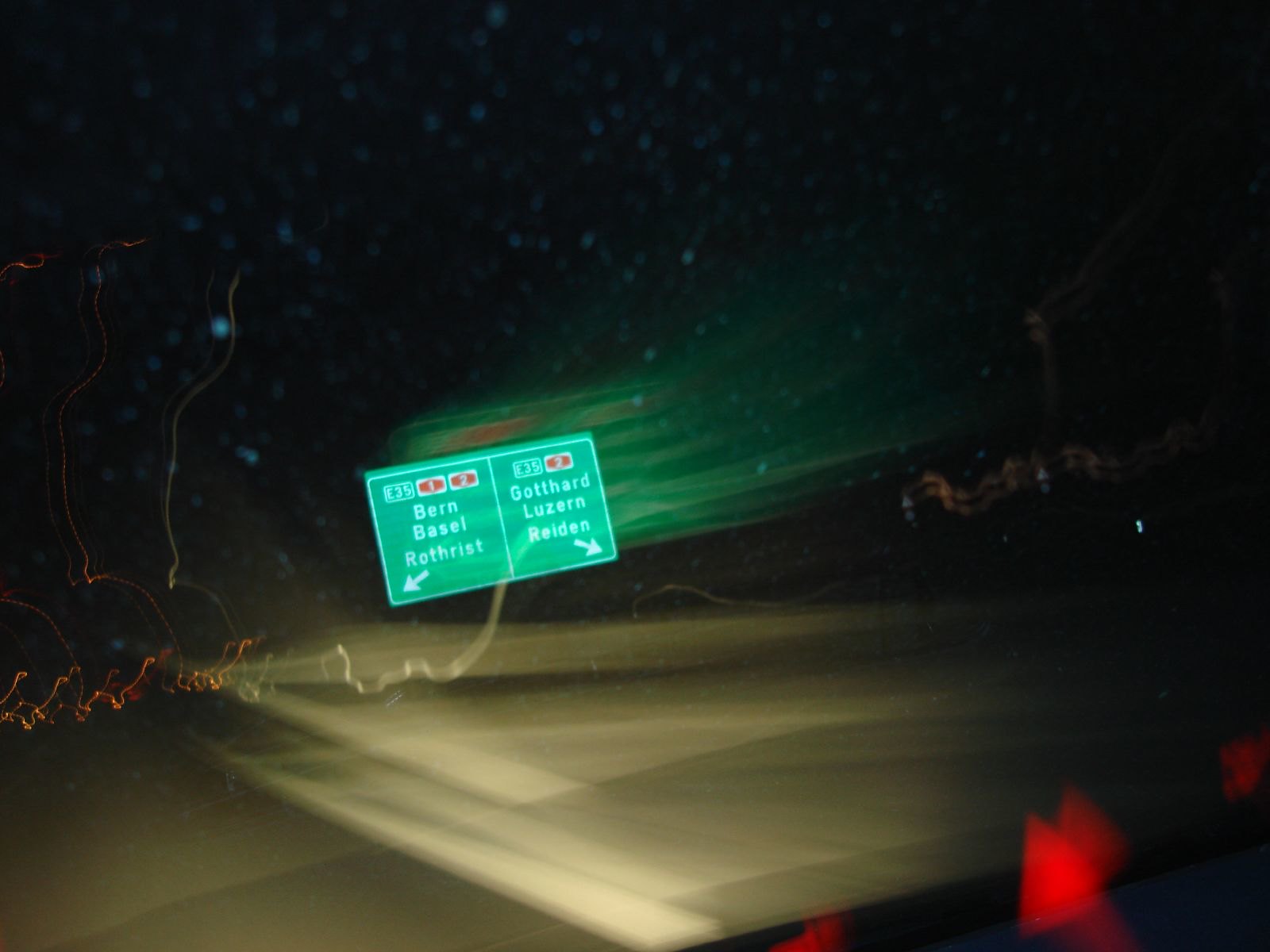A nighttime, blurry photograph taken from inside a vehicle features a partially illuminated dashboard in the bottom right corner with various lights lit up. The image captures a green road sign, which appears slightly tilted and is divided into two sections. The left section directs travelers towards "Burn Basil" with an arrow pointing left, accompanied by the designation "E35." Positioned above the E35 is a white rectangle with red ovals marked "1" and "2." The right section of the sign points towards "Godhard Luzerin Reden" with an arrow indicating the right direction, also marked with "E35." Above the E35 on this side, there's a white rectangle featuring a red oval marked "2." The scene is dim, adding to the mysterious ambiance of the nocturnal journey.